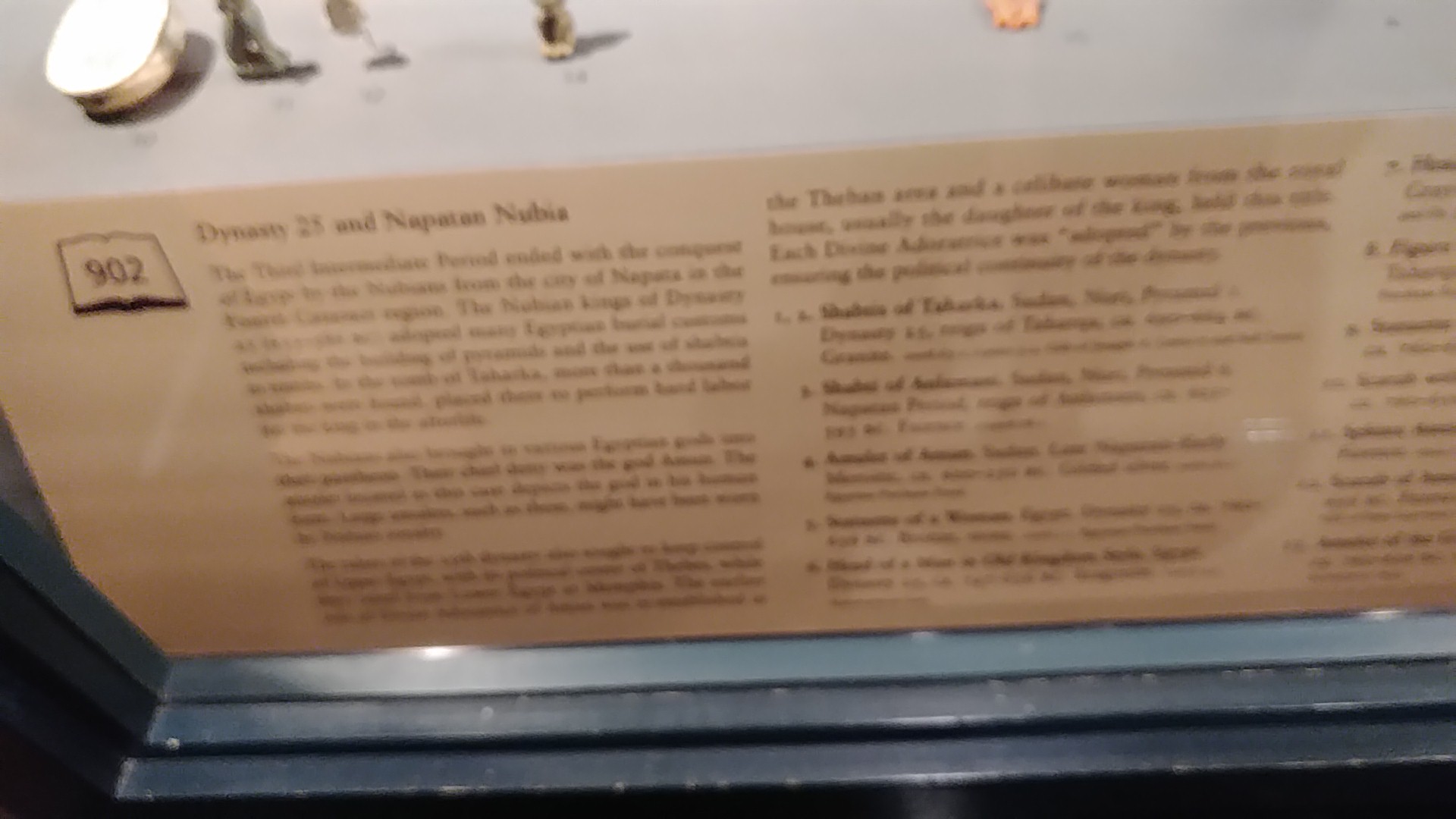In this image, we observe a display through what appears to be a glass partition or window. The display features a collection of numbered objects placed on a white shelf at the top. To the left of this shelf, there is a light illuminating the scene. Below the shelf, there is a section of text written in black on light brown or beige paper. Although the text is slightly out of focus, several details are discernible: it includes the number "902," and references to "Dynasty 21," "Dynasty 23," and "Napatan Nubia." The text seems to contain a header followed by a couple of paragraphs that describe the objects in the display, potentially numbering and titling them with bold text. At the bottom of this textual section, there appears to be some sort of bench or wooden structure, adorned with small blue bars, some of which are faintly illuminated.